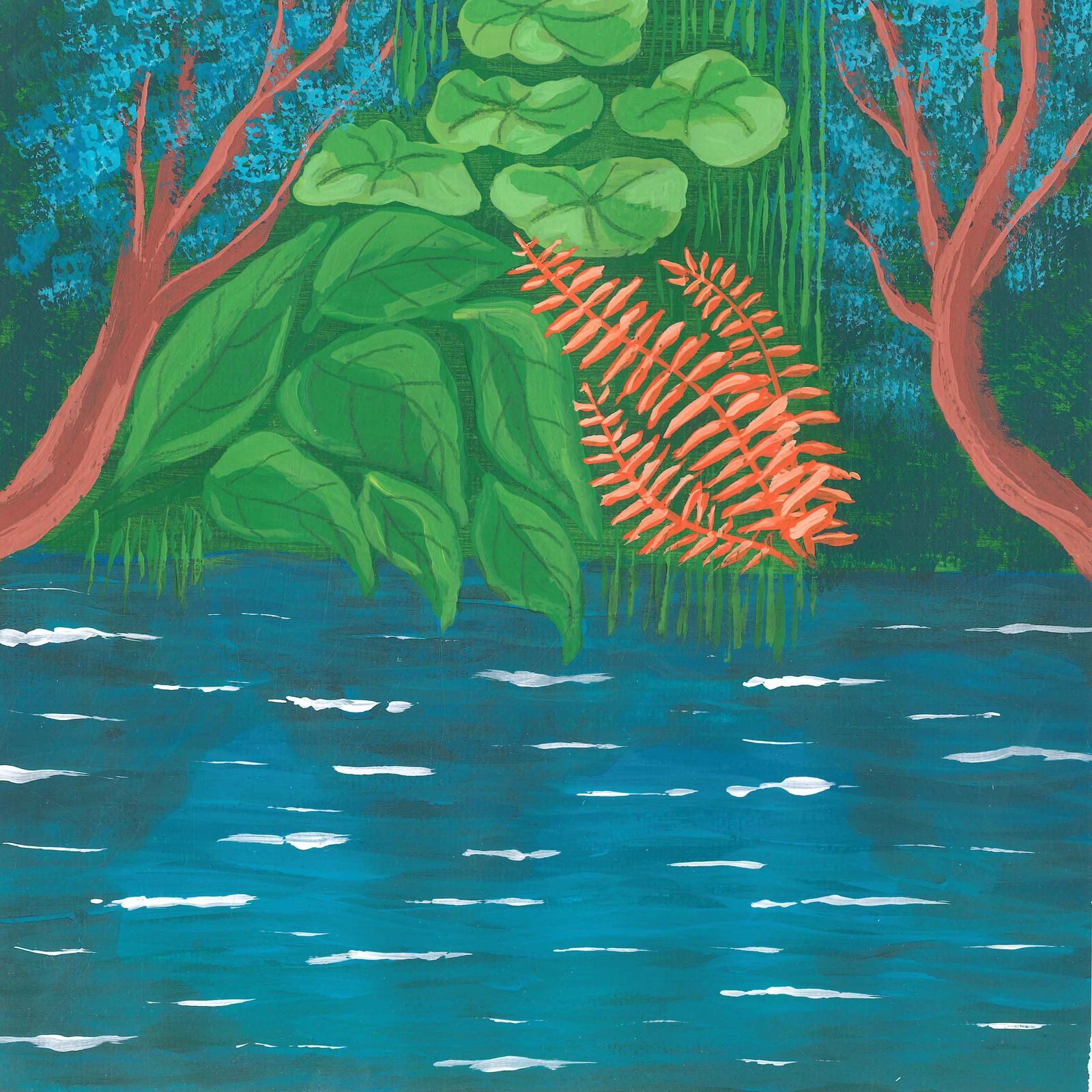This image is a detailed painting of a lush, watery jungle scene. The bottom half of the composition features aqua blue water accented with small, white wave reflections suggesting motion. Rising from either side of the water are two prominent tree trunks with light reddish-brown bark, adorned with delicate blue flowers. Flanking these trees are a myriad of plant life; giant, vibrant green leaves extend from the left and right, with some dipping into the water. Additionally, long, stringy green foliage resembling lichen or vines drape gracefully between the trees, enhancing the jungle atmosphere. Lower in the image, large golden fronds emerge vertically along the riverbank. More plants, including a distinctive reddish-orange fern with triple stems, and a backdrop tinged with shades of blue and green, complete the vivid scene.